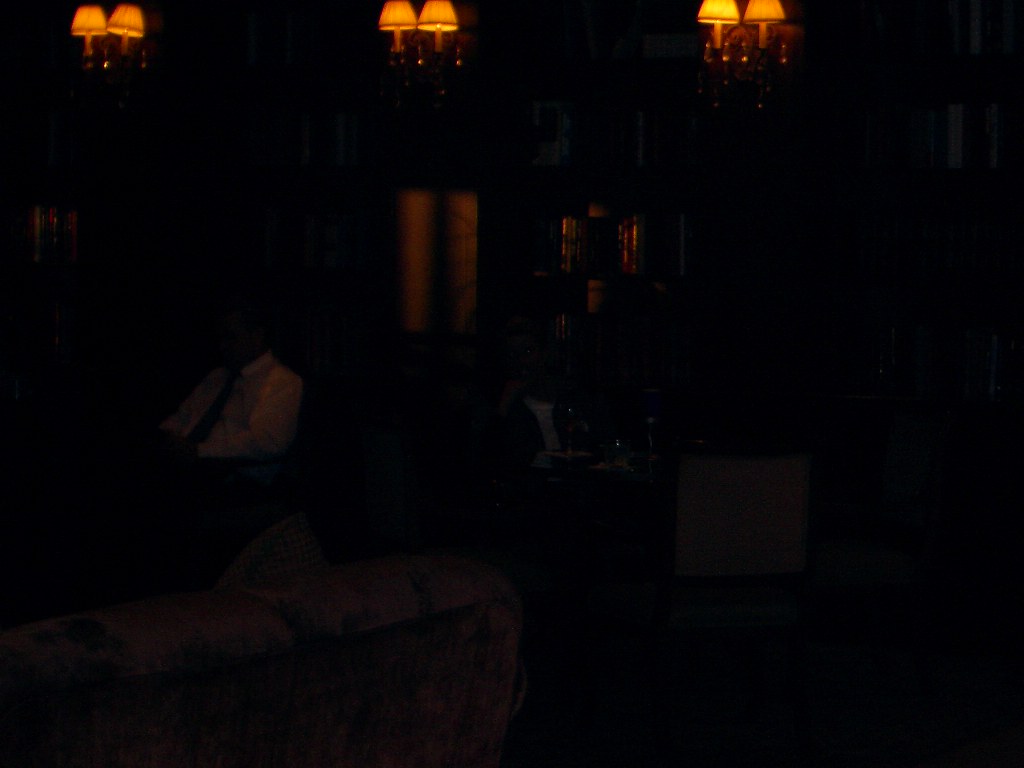This photograph is a dimly lit indoor scene characterized by deep shadows and sparse illumination. The upper left section near the middle of the top edge and extending towards the right features a series of sconces affixed to the walls. These sconces boast off-white lampshades, arranged two per fixture, imparting a soft elegance. Beneath these lampshades, gold vertical bars extend downward, adding a touch of opulence to the scene. To the right, a subtle bronze-toned lighting element comes into view, contributing to the ambient glow. In the lower left corner, the faint outline of what seems to be a face with dark hair emerges from the darkness, shrouded in mystery. The majority of the photograph remains enveloped in blackness, leaving much to the viewer's imagination.